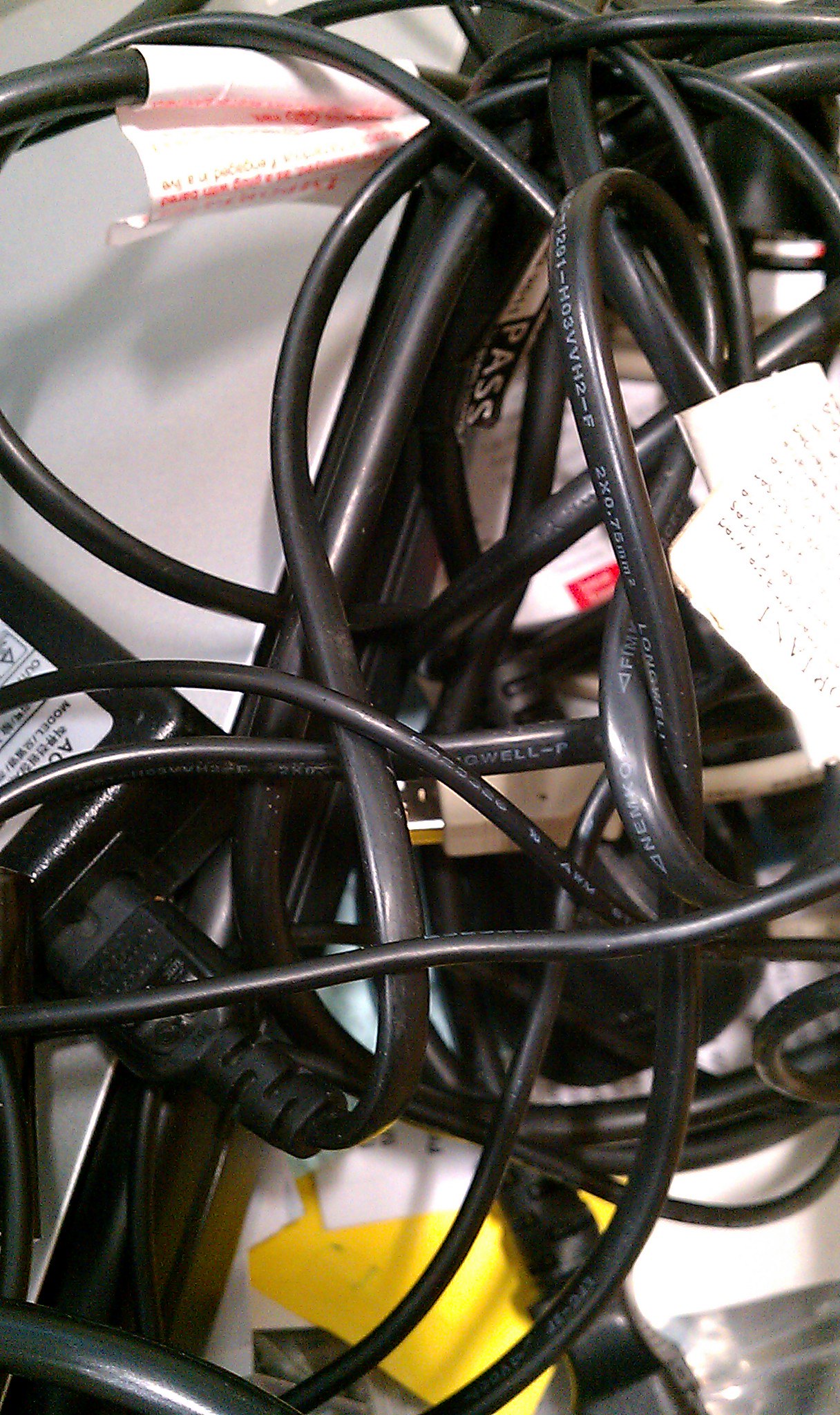The image features a tangled and intertwined mass of black wires sprawled across a surface that appears to be indoors, possibly in someone's computer room or a drawer. The background is mostly white, with various receipts, papers, and envelopes interspersed throughout the scene. Notable elements include an AC adapter on the left side, alongside several plugs connected to it, with wires extending outward. Among the wires, there are labels, some printed in white text directly on the wires, and others attached as white paper tags. A yellow object, likely a triangle, is visible at the bottom of the image. The overall array of objects, which seems to include electronic equipment and possibly a laptop, is haphazardly arranged, with no particular item centered in the photo. The predominant colors in the image are black, white, gray, orange, red, and yellow.